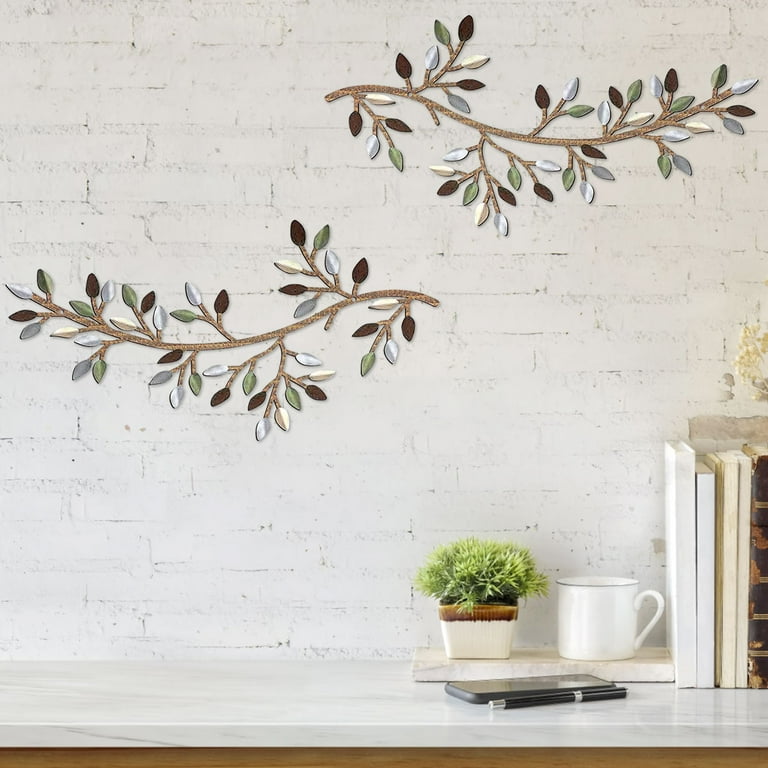The photograph features a white-painted brick wall with the outlines of the bricks still visible, creating a textured background. Two pieces of metallic branch artwork adorn the wall, with leaves in shades of silver, gold, deep brown, and green, positioned towards the center left and the top right of the image. In front of the wall is a white marble countertop, accented by a brown wooden trim below it. On the right side of the countertop, a smartphone rests next to a sleek black and silver pen. Behind the smartphone is a small plant in a cream-colored and brown square pot. To the right of the plant sits a plain white coffee mug. Further to the right, five books, varying in tones of white and cream, are standing upright, acting as a visual anchor on the countertop. The combined elements create a harmonious and visually appealing arrangement.